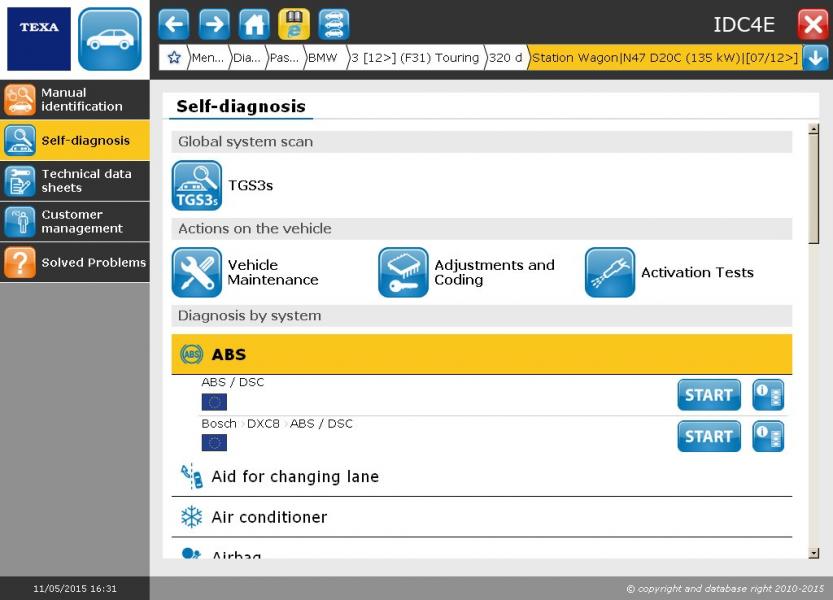The screenshot depicts a user interface from a website called Texa. In the top left corner, the Texa logo is enclosed in a navy blue box. Adjacent to the logo, to the right, is an image of a car situated within a light blue box with rounded corners. Below these elements is a vertically oriented menu bar featuring a list of options, each with a black background and an icon beside them. The menu items are as follows: "Manual Identification," "Self-Diagnosis" (highlighted in yellow), "Technical Data Sheets," "Customer Management," and "Solved Problems."

The primary focus of the image is on the right-side pane, which occupies the majority of the screenshot. This area shows a browser window with a black header containing several tabs and icons, though the tabs are partially condensed and unreadable. The upper portion of the content area on this webpage displays the title "Self-Diagnosis" on the top left, right beneath the tabs, underlined in blue.

Below the title, the page is divided into three sections, each highlighted in gray:

1. **Global System Scan**
   
2. **Actions on the Vehicle**
   - This section includes three icons labeled:
     - Vehicle Maintenance
     - Adjustments and Coding
     - Activation Tests

3. **Diagnosis by System**
   - The first row, highlighted in yellow, is labeled "ABS" and features a "Start" button on the far right.
   - The next two rows display the label "ABS DSC" with a European Union tag and a "Start" button on the far right.
   - The second row specifically mentions "Bosch DX C8 ABS-DSC," also with an EU tag and an accompanying "Start" button.
   - Below these are three more rows: "Aid for Changing Lanes," "Air Conditioner," and "Air Bag."

This detailed view provides an intricate overview of the self-diagnosis functionality embedded within the Texa website, highlighting various diagnostic options and interactive elements.